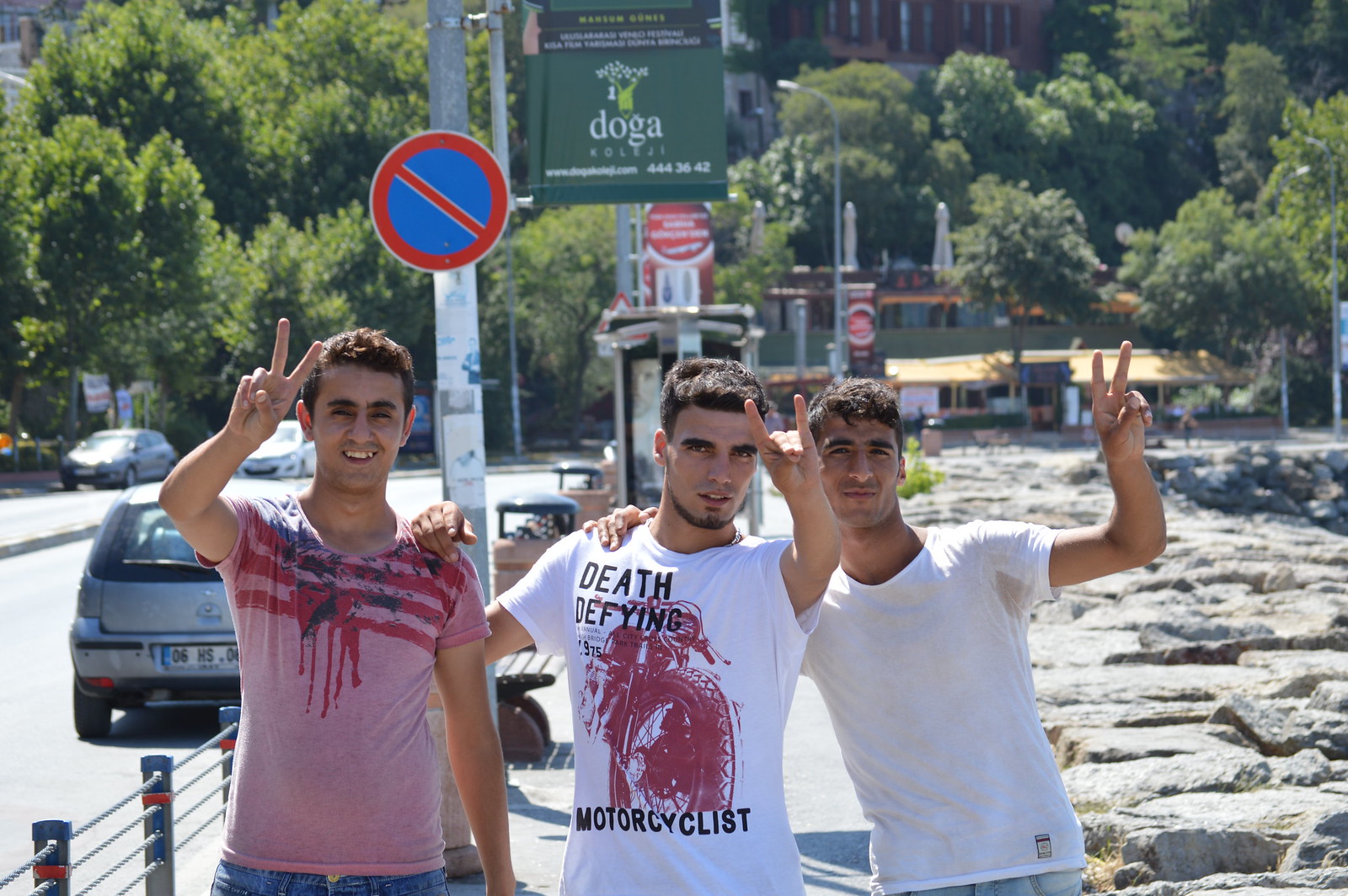In this vibrant photograph, three friends are striking playful poses for the camera, each expressing their unique personality through hand gestures. The first individual, donned in a bright pink shirt, flashes a peace sign, symbolizing harmony and goodwill. The second friend, in a white shirt emblazoned with the words "Death-Defying Motorcyclist," confidently displays a bull sign with his fingers. Meanwhile, the third companion, also in a clean white shirt, joins in the fun by holding up a peace sign.

The trio stands on a rocky path that leads down to a road, surrounded by the lush greenery of trees in the background, hinting at a picturesque outdoor setting. Overhead, a sign reads "Doga," accompanied by another sign bearing a circle with a slash through it, possibly indicating a prohibition. The carefree spirit and camaraderie of the friends, captured in front of this intriguing backdrop, make for an engaging and lively snapshot.